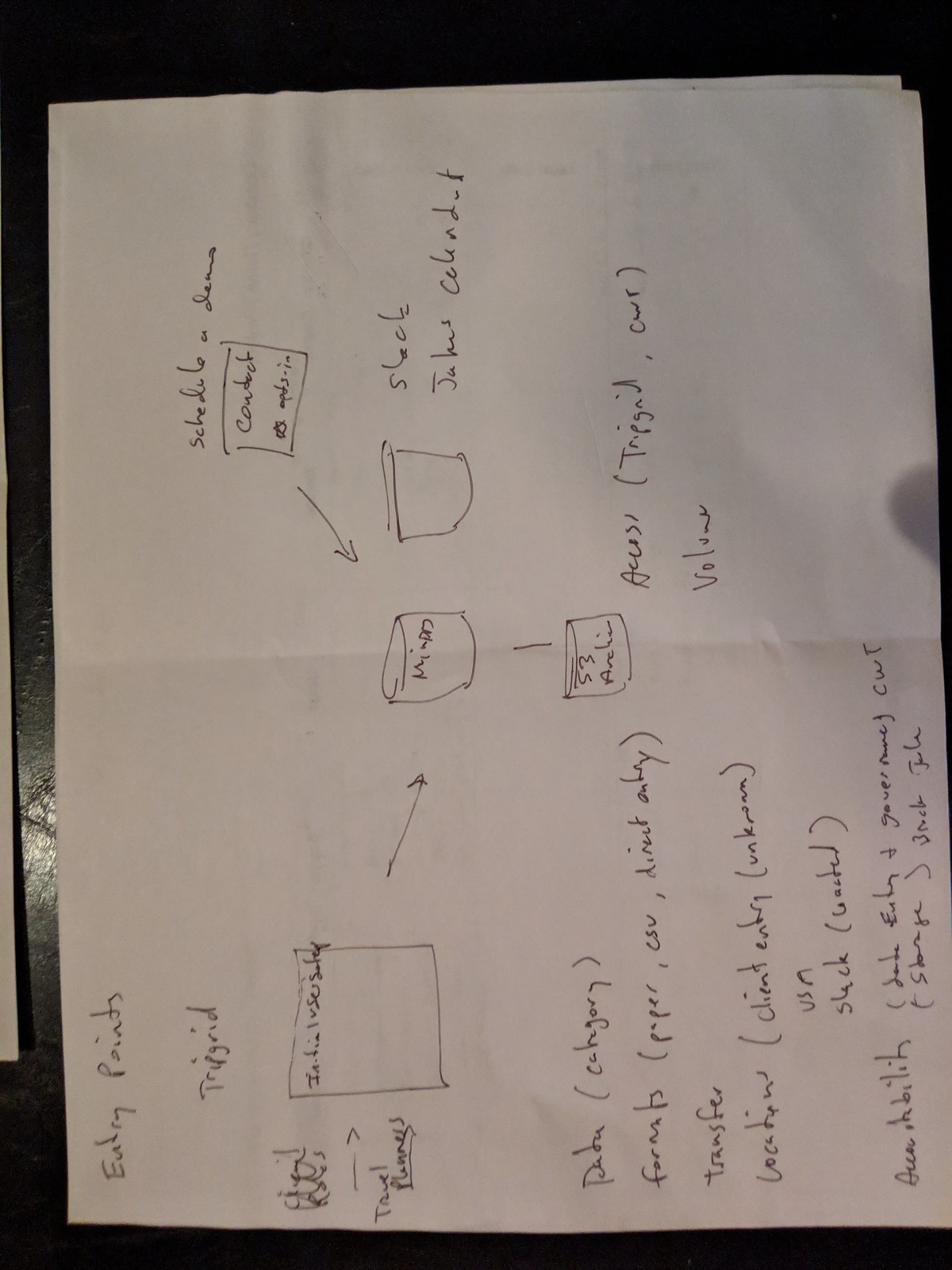The image features two sheets of white paper set against a sleek, black, presumably leather surface. The top sheet, which is central to the image, shows visible creases from being folded and then unfolded. Although partially obscured, the second sheet lies directly beneath it. 

The text covering the top sheet is challenging to decipher, but it appears to feature a diagrammatic representation of early painting techniques. This diagram includes a series of shapes and arrows: a square, an arrow leading to a cylinder, another cylinder beneath it, and another square with an arrow pointing to the same central cylinder, suggestive of a process flow. Additional text is located in the bottom right corner of the image—actually on the bottom left of the paper—containing several parenthetical notes and more illegible writing continuing down to the bottom of the page. The image is distinctly oriented vertically, giving a top-down view of these elements.